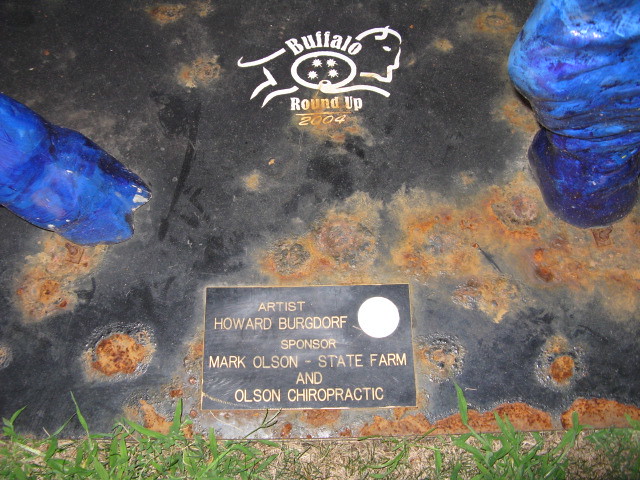The image depicts an outdoor artistic statue, seemingly part of a public exhibition. Set against a grassy area, it features two lumpy, blue ceramic pieces on the top corners, painted in various shades of blue and accented with touches of purple. The centerpiece is framed by a weathered, rusted black metal base, giving it an aged and somewhat neglected appearance. Prominently, in the top center, there's a logo with a buffalo illustration accompanied by the text "Buffalo Roundup 2004" in white letters on a dark background. Below this, a gold-lettered plaque provides details about the artwork, stating "Artist: Howard Bergdorf, Sponsor: Mark Olson State Farm and Olson Chiropractic." This combination of elements suggests a commemorative piece celebrating the Buffalo Roundup event from 2004.